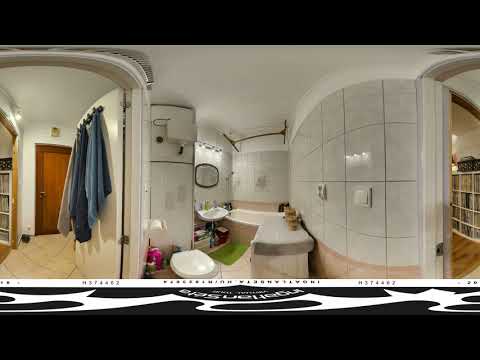The image prominently showcases a central bathroom with white rectangular tiled walls, evoking a chill and laid-back cruise ship ambiance. At the lower left, a one-piece toilet is visible. The countertop across the room is white with a grayish covering, adorned with various objects. In the background, there's a bathtub beside a sink, under which a brown wastebasket is placed. Above the sink is a mirror, and in front of it lies a lime green rug. To the left is an adjoining room featuring garments hanging and a brown door leading out. To the right, another room has a brown hardwood floor and a white cabinet with multiple shelves, with a decorative item on top. The entire scene, captured with a fisheye lens, also depicts the roof as predominantly white, and it incorporates black and white horizontal lines along the top and bottom, emphasizing the comprehensive 360-degree view of the three interconnected rooms.